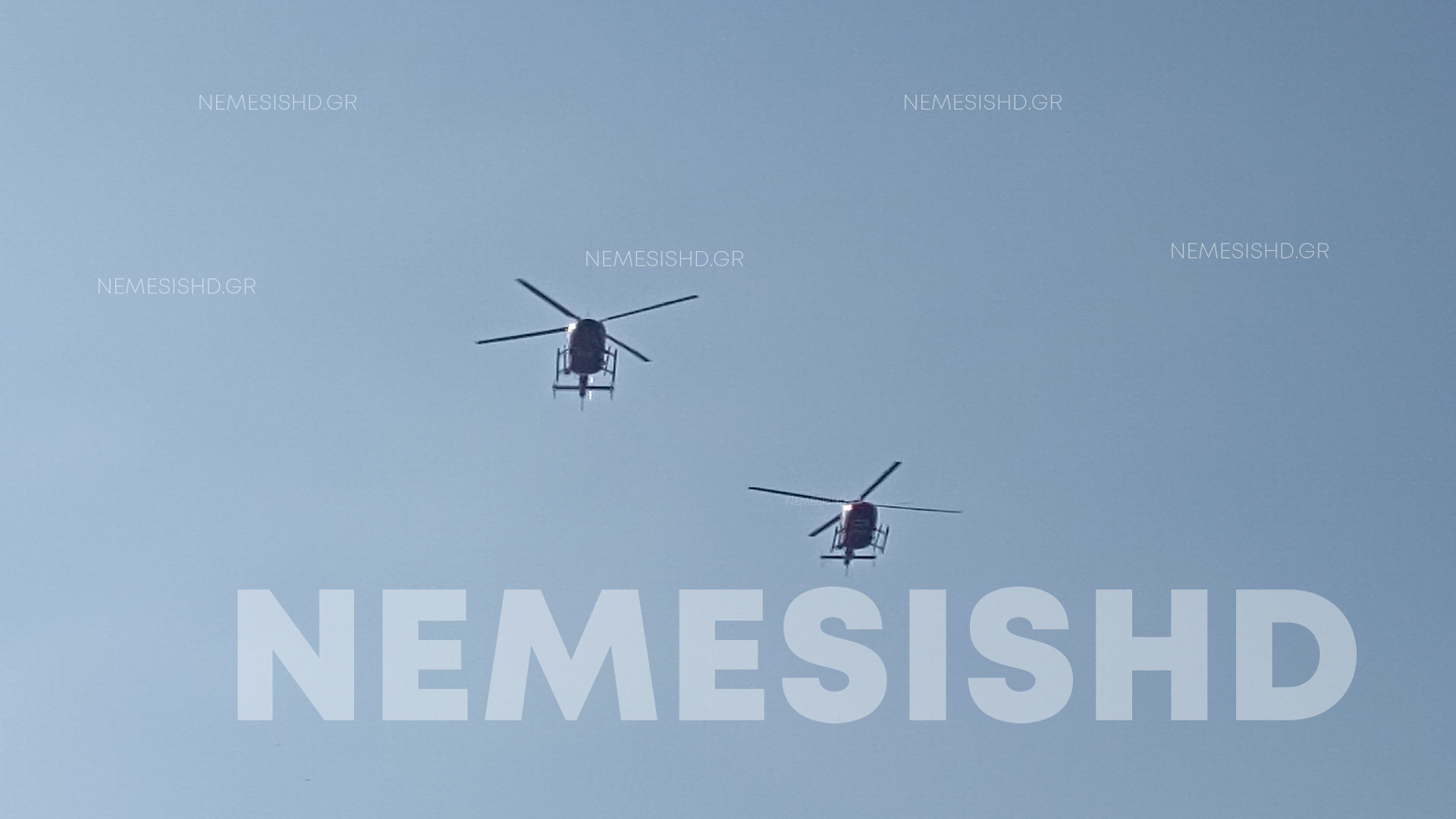A stunning photograph captures a pair of helicopters soaring across a clear, blue sky. The sky is uniformly blue, with no visible land or background, focusing attention entirely on the helicopters. Positioned slightly apart, one helicopter is located higher up on the middle left, while the other is lower and toward the middle right. Both helicopters, which are black and feature four rotors each, are flying relatively close to each other, suggesting they might be operating together. No specific logos or details are discernible due to the distance. A distinct watermark dominates the image, with "Nemesis HD" prominently displayed in large, grayish-blue letters at the bottom. Additionally, five smaller inscriptions reading “Nemesis HD” and accompanied by the ".gr" domain, are scattered across the photo, reinforcing the watermark. Bright sunlight creates a subtle glare on the left side of the scene, adding a touch of dynamism to the photo.